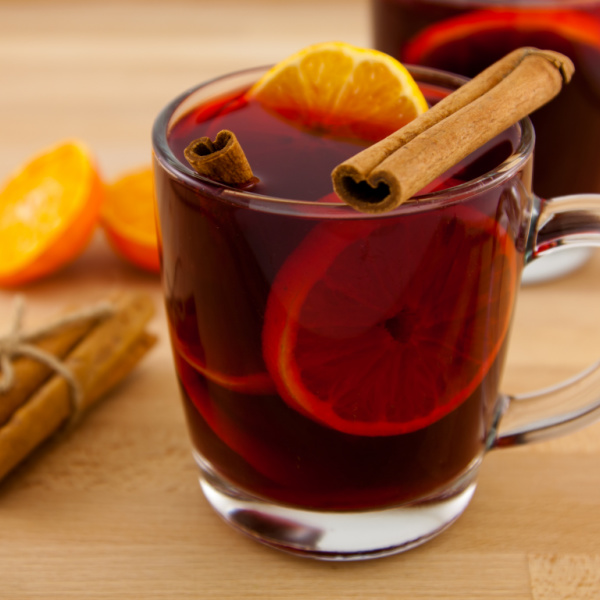In this detailed square-format color photograph, a clear glass mug filled with dark reddish-brown tea takes center stage. The handle of the mug is oriented to the right side of the image. Floating within the tea are several slices of vibrant orange, adding a splash of color and freshness. On top of the mug lies a cinnamon stick, while another is inserted into the drink, adding a rustic and aromatic touch.

The mug is situated on a light brown, wood-textured surface. To the left of the glass, there is a neatly tied bundle of cinnamon sticks, secured with beige twine, emphasizing the aromatic theme of the setting. An orange, sliced in half, rests further to the left, complementing the orange slices inside the mug. 

In the background, on the top right, you can partially see another mug of tea, hinting at a cozy setting possibly prepared for more than one person. There are no people or text in the image, keeping the focus on the richly detailed and beautifully arranged ingredients and the inviting mug of tea.